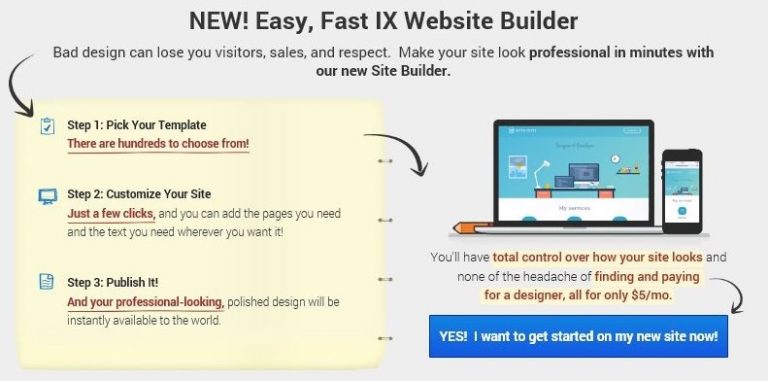**Descriptive Caption:**

The screenshot features a gray background with a comprehensive step-by-step guide for using a new, user-friendly site builder. At the top, bold text highlights how bad design can negatively impact your website by losing visitors, sales, and respect. The guide then emphasizes the simplicity and efficiency of the new site builder, claiming that you can create a professional-looking website in minutes.

**Step 1**: Choose from hundreds of templates (highlighted in red).

**Step 2**: Customize your site with just a few clicks, adding necessary pages and text wherever you desire.

**Step 3**: Publish your site, ensuring that your polished design is instantly available to the world.

The diagram includes visuals of a laptop and a cell phone, underscoring that users will have "total control" over their site's appearance without the typical headaches of hiring and funding a designer—all for only $5 a month ($5/mo.).

A blue rectangle at the bottom prompts users with a call to action in white text: "Yes! I want to get started on my new site now!"